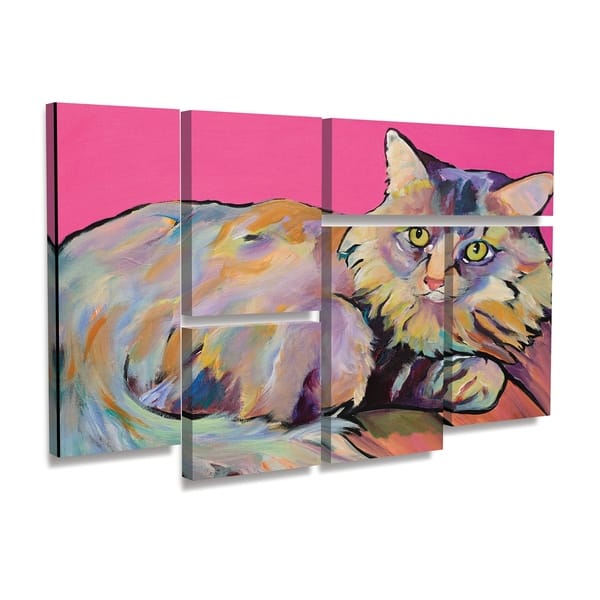The image is an intriguing painting of a cat, made up of six distinct panels arranged closely together, reminiscent of a puzzle. The combined panels depict a gray Maine Coon-type cat, with splashes of orange, black, blue, and purple throughout its fur, giving it a dreamlike quality. The background is a vivid fuchsia pink. 

The layout of the panels is as follows: On the far left, there's a tall rectangular panel showcasing mostly the cat's back and tail. To the right, there are two canvases stacked vertically—a rectangular one on top and a square below it—forming the main body of the cat. At the top right, a horizontal rectangular panel features the cat's ears. Beneath this panel are two vertical rectangles; the left one is taller than the right, and together they display the cat's face and front paws. The cat has striking greenish-yellow eyes and a light pink nose, and it appears to be sitting on its side within the composite image, which floats against the white space surrounding the panels.